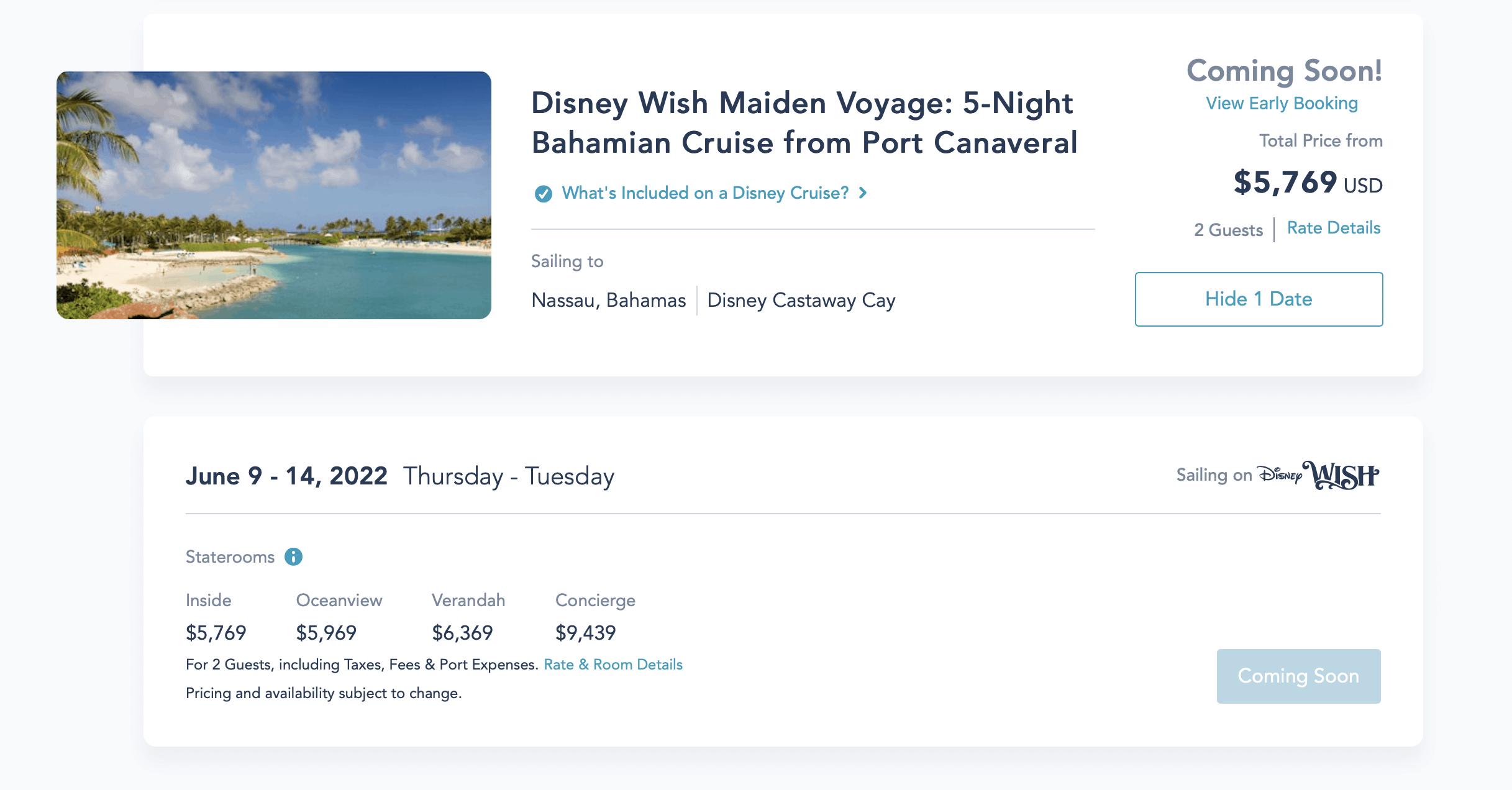Here is a detailed and cleaned-up caption for the image described:

---

The image advertises a Disney Cruise, featuring a serene turquoise ocean that transitions into a tranquil lagoon with white sandy shores, beneath a clear blue sky. Text overlay indicates "Disney Wish: Maiden Voyage - 5-Night Bahamas Cruise from Port Canaveral." Below this is a blue-arrowed button labeled "What's included with the Disney cruise."

Additional details include:
- Destinations: Nassau, Bahamas, Disney Castaway Cay (with "Coming Soon" notes and a link for early booking).
- Pricing: Starting from $5,769 USD for two guests.
- Rate breakdown:
  - Inside cabin: $5,769
  - Oceanview cabin: $5,969
  - Verandah cabin: $1,369
  - Concierge: $9,439
  (All prices include taxes, fees, and port expenses).
- Dates: June 9th through 14th, 2022 (Thursday to Tuesday).
- Voyage: Sailing on Disney Wish.

There are interactive elements like a "Hide 1 Detail" button, and "Rates and Room Details" link showing further information. 

---